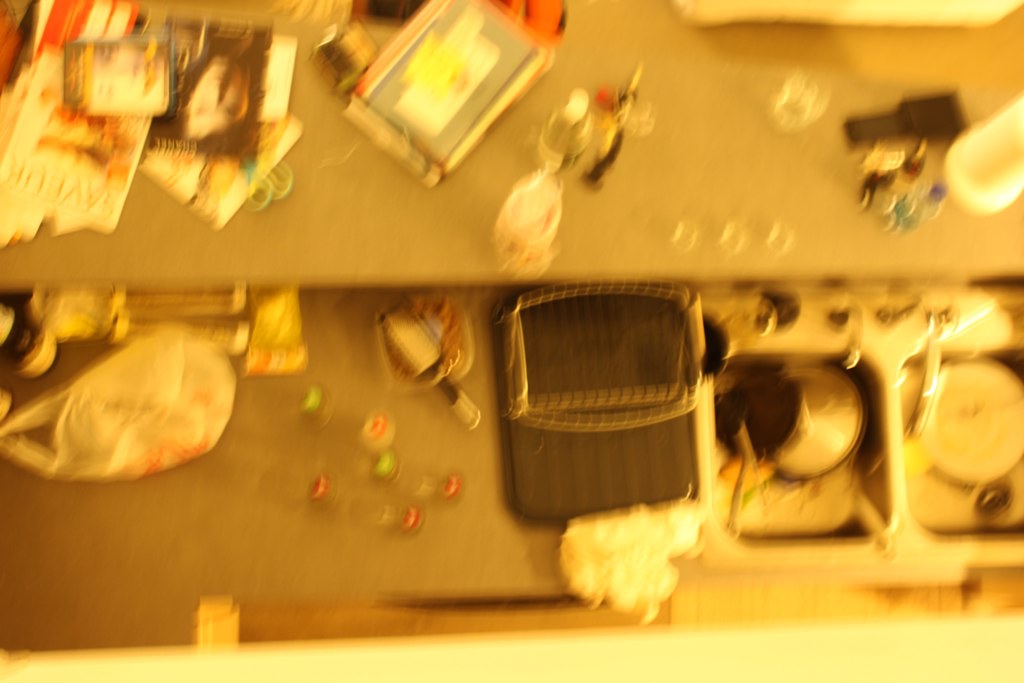This image provides an overhead view of a significantly blurred kitchen counter, making detailed identification of items difficult. The scene captures a range of everyday objects scattered across the surface, exemplifying a functional but cluttered space. 

On the left side, a dense collection of assorted items, potentially including books, magazines, kitchen-related paperwork, or small gadgets, suggests that this area serves multiple purposes beyond cooking. The clutter here is particularly intense, indicating a busy household environment.

In the center of the image, there's a prominent dark-colored tray or shallow container. Surrounding this central object are several small, round items, which might be fruits or small kitchen tools, giving a glimpse into the daily culinary activities performed here.

The right side of the counter holds more orderly arranged objects, including glasses and dishes, providing a contrast to the chaotic nature of the left side and central area. This section appears to be more organized, demonstrating an attempt to maintain some order amid the overall messiness of the kitchen space.

Despite the blur, the image captures a snapshot of a bustling kitchen, rich with details that hint at the diverse activities and items that populate this household's daily life.